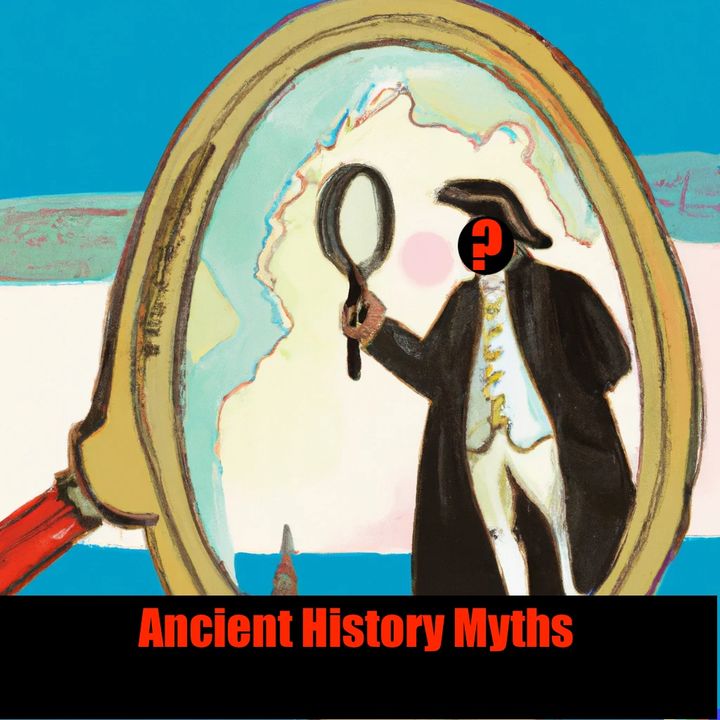This illustration, possibly created with markers or crayons, vividly captures the essence of ancient historical myths as referenced by the bold red text on a black border at the bottom. At the heart of the drawing is an intricately detailed magnifying glass with a gold rim and a distinctive red handle. Standing inside this magnifying glass is a mysterious figure, garbed in elaborate colonial-era attire reminiscent of George Washington, complete with a gold-embroidered vest, gold buttons, and tight white pants. This gentleman, donning a cape and a distinctive tricorn hat, holds another magnifying glass while his face is obscured by a black circle marked with a red question mark, heightening the intrigue. The background features a map-like texture with alternating turquoise, red, and white stripes, adding depth to the scene, which extends into a blue sky beyond the lens. The artwork employs a rich palette, including primary colors such as blue, tan, red, green, black, yellow, and white, seamlessly blending them to capture both historical reverence and artistic mystery.